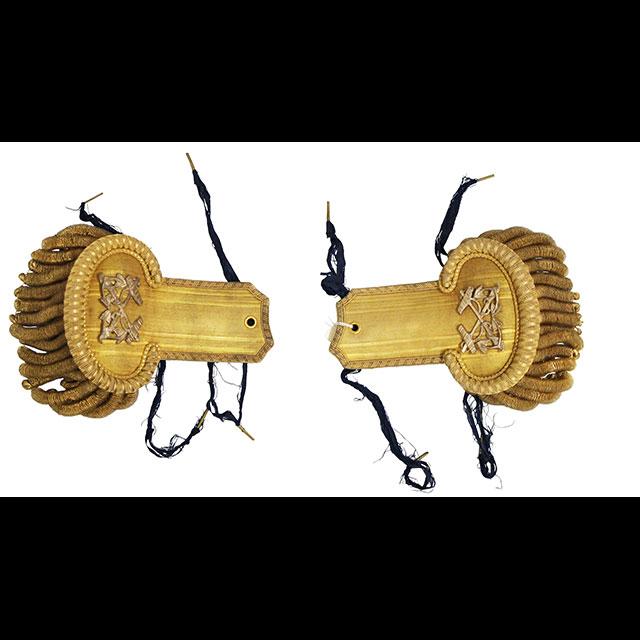The image displays two identical objects placed side by side on a white background, each with a light brown wooden handle oriented towards the center. These objects feature an oval-shaped extension with intricate raised designs in the middle, surrounded by beading. The objects appear to be highly ornate, golden-colored, and possibly used for decorative purposes, such as shoulder decorations in the military.

Each object has a series of thick, finger-like projections extending below the oval, resembling a brush, although the ends appear soft and pliable. Black stringy material is seen emerging from both ends of the handle bases and the lower ends of the oval extensions. In the middle of both handles, there is a small hole, with the right one showing some white string coming out of it. Additionally, frayed black fabric pieces can be observed, suggesting these might have been sewn onto clothing at some point.

The entire scene is bordered by thick black bars at the top and bottom of the image, approximately an inch in width, providing a stark contrast to the central composition of the ornate objects.